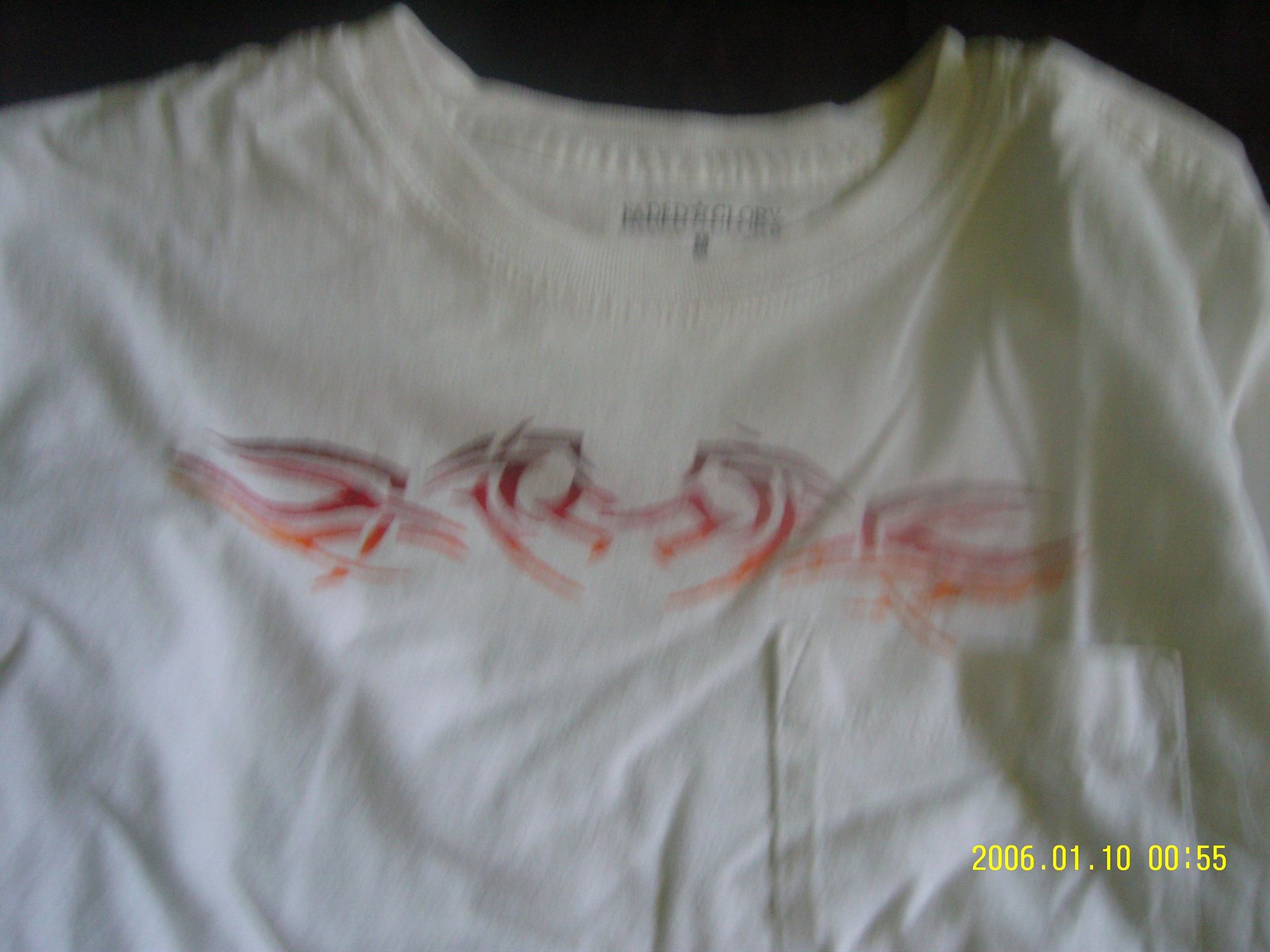This blurry, close-up photograph, possibly taken indoors using an old digital camera or phone, features the top part of a heavily wrinkled, white round-neck t-shirt. The t-shirt has a pocket on the left breast and a distinctive geometric line design across the chest in shades of orange, red, and maroon, with the center of the design resembling a heart or a tribal symbol. The tag near the collar reads "Faded with a Star, Glory" in black text, and denotes the shirt size as medium (M). In the bottom right corner of the image, a yellow timestamp reads "2006.01.10 0055," indicating that the photograph was taken at five minutes to one in the morning. The background of the image is black, making the details on the t-shirt stand out despite the poor image quality.